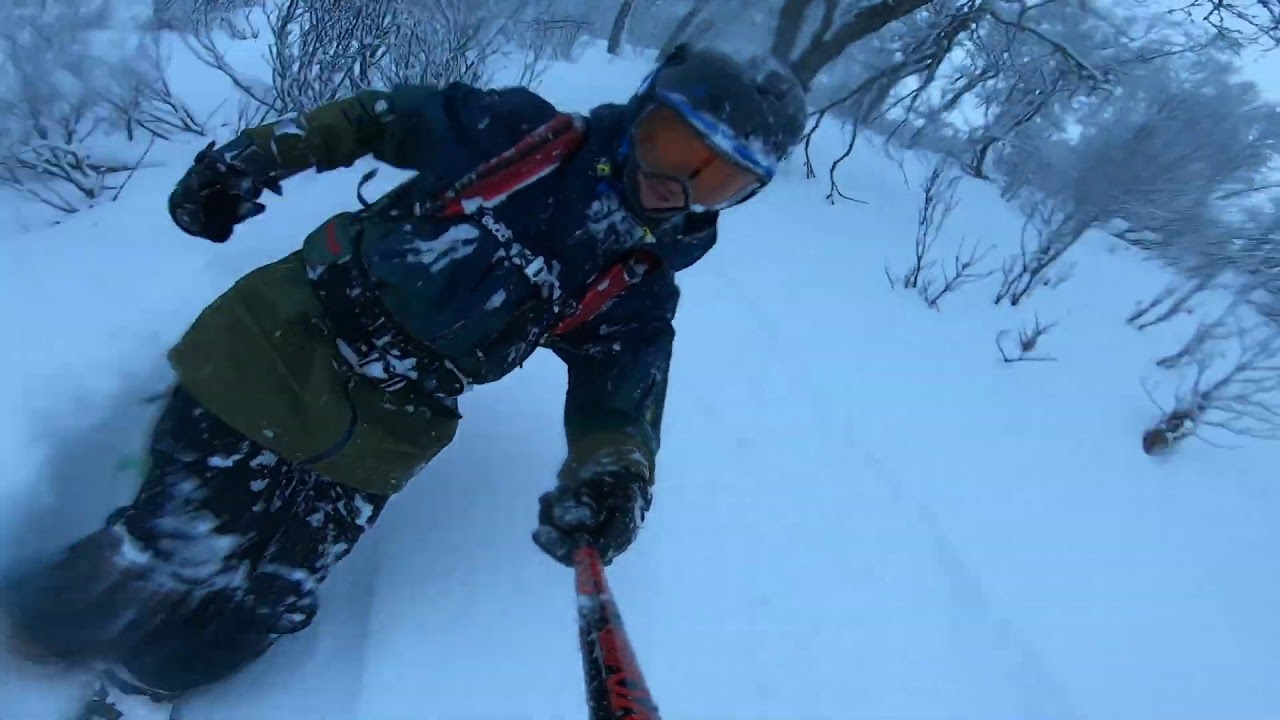This photograph captures a dynamic moment of a skier taking a selfie on a snow-covered mountain. The skier, equipped for winter, is wearing a blue jacket, blue pants, and a khaki layer in the middle. He is also donned in essential protective gear including a helmet with orange-tinted goggles. The snowy conditions are evident as snow clings to his attire. In one hand, he holds a black and red selfie stick to capture this high-spirited moment. Surrounding him is a picturesque winter landscape with dry, leafless trees dotted throughout the deep snow, highlighting the serene and frosty atmosphere. The skier's backpack, suggested by the visible red straps over his shoulder, adds functionality to his vibrant ensemble.